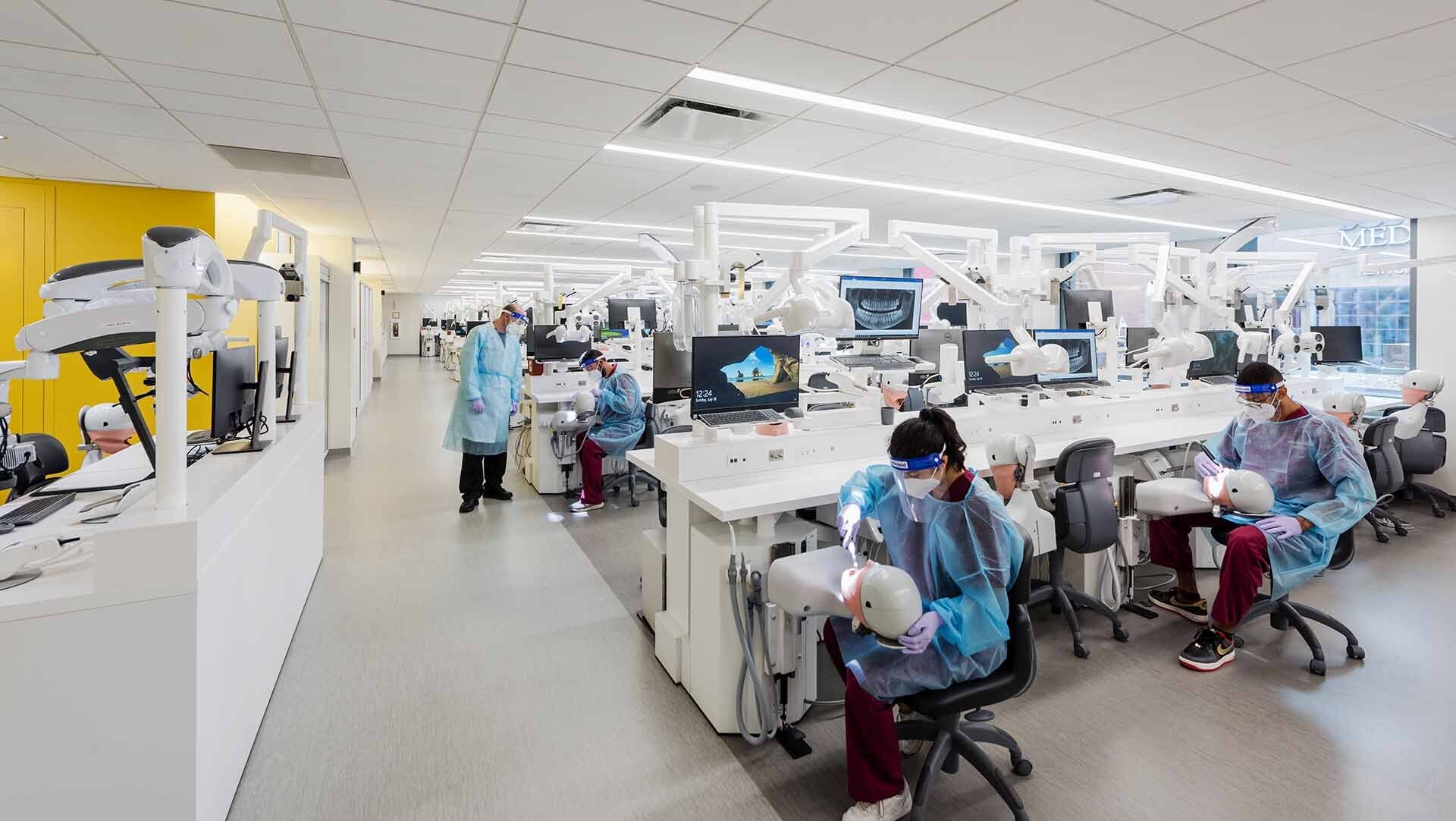The image depicts a modern dental school laboratory with a spacious, well-lit room featuring tiled ceilings and built-in strip lighting. In the foreground and mid-ground, several students, likely dental students or dental hygienists in training, are actively engaged in practical exercises. They are dressed in blue medical scrubs, N95 masks, plastic gloves, and overgarments. Each student is working on a dental mannequin with an open mouth, indicative of dental practice procedures.

The classroom is equipped with numerous desks, each featuring computer monitors and various dental apparatus typical in a dental lab setting. The setup includes multiple rows of workstations with dental trays and articulated arms, all arranged neatly across the room. On the left side of the image, there's a walkway adjacent to a yellow wall with a couple of doors, adding a touch of color to the predominantly white and sterile environment. 

Towards the center of the image, a supervising professor, also dressed in similar protective attire, is seen leaning over to assist one of the students. The overall ambiance is that of a highly organized and meticulously maintained educational space, designed to facilitate hands-on learning and skill development in dentistry.